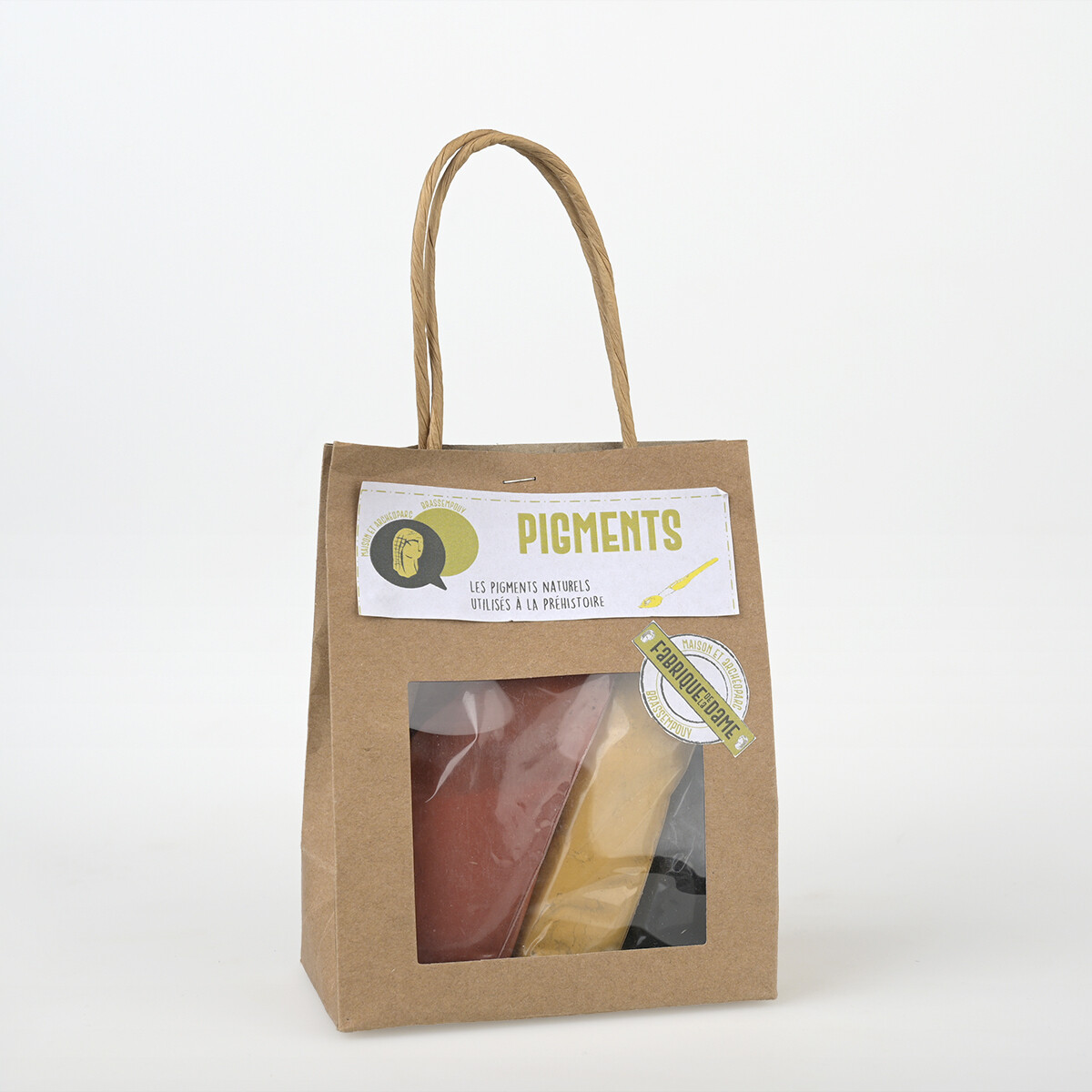In this photograph, there is a brown, heavy-duty paper shopping bag featuring a pair of sturdy looped paper handles at the top, which is stapled shut. The bag sits on a white, featureless surface. Prominently displayed on the bag is a label with text in a yellowish-green color that reads "Pigments." Below this, there are several lines of French text: "Les pigments naturels utilisés à la préhistoire" and "Fabrique de la Dame." The bag includes a rectangular cut-out with a transparent plastic cover that allows a clear view inside. Through this window, you can see three smaller bags containing powdered pigments in distinct colors—red on the left, yellow in the middle, and black on the right. Additionally, there is a white rectangular piece of paper stapled to the outside of the bag with "US Pigments" on it, accompanied by two comic book-style word bubbles in light yellow and gray.